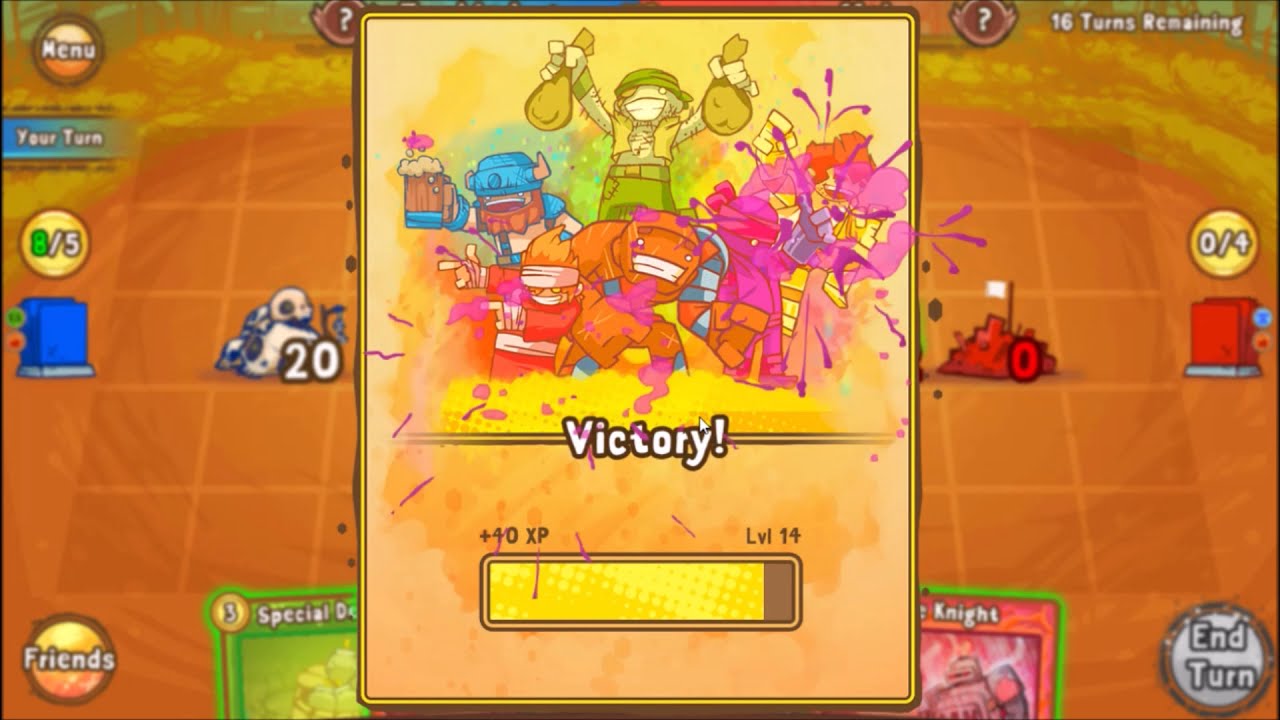The image is a detailed screenshot from a colorful, cartoonish video game. Dominating the foreground is a large vertical rectangle, reminiscent of a card, stretching from the top to the bottom of the screen. This rectangle features a tan background populated with vibrant cartoon characters in a festive scene; one character holds two bags of money while another raises a beer, all suggesting a celebratory atmosphere.

Prominently displayed in white, bold letters at the center of this card is the word "Victory!" accompanied by an exclamation mark. Below this, a nearly full, horizontal yellow progress bar indicates player advancement, with "+40 XP" on its left side and "Level 14" on the right.

The background of the image is filled with an orange and yellow hue, creating a warm, inviting ambiance. The entire screen is bordered with various graphical user interface elements: "Menu" in the upper left, "16 turns remaining" in the upper right, "Friends" inside a circle in the lower left, and "End Turn" on the bottom right. The background surface appears to be composed of tiles viewed from an angle, and the bottom edge of the screen shows additional cards or elements, completing the immersive gaming environment.